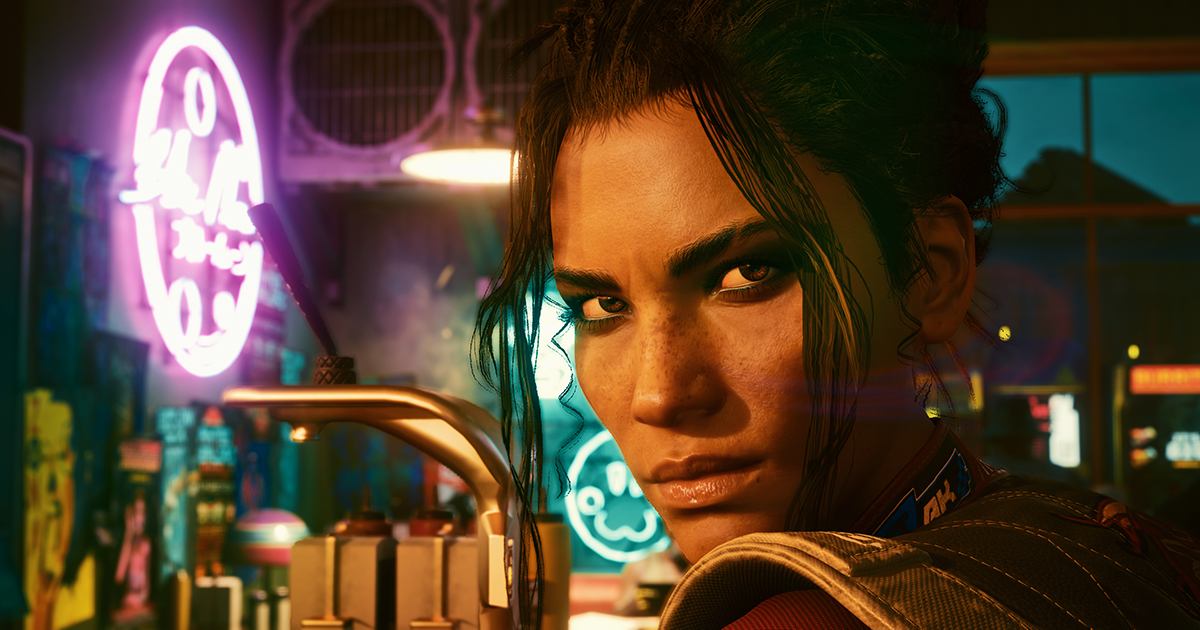The image is a digitally-generated depiction of a young woman, approximately 25 years old, named Manfalkenborn. She has short black hair partially pulled back, with some strands falling across her face. Her dark eyebrows and expressive dark eyes give her a superhero-like appearance. 

Manfalkenborn is seen wearing a brown, military-style vest or armor over her shoulders, which resembles a backpack. The background appears to be a bar, as suggested by the presence of various neon signs and taps. One neon sign has a white base with a pink glow, while another has a green glow, but neither are readable. 

Above, there are big fans and lights hanging from the ceiling, adding to the intricate detailing of the surroundings. Behind her, through a partly dark, dark-blue window, there is a view of a mountain, some shiny and golden containers, and an orange sign, though its text is also unreadable. The background is filled with a blend of colors including white, pink, black, blue, green, yellow, brown, and orange, which contribute to the vibrant yet somewhat surreal atmosphere of the image.